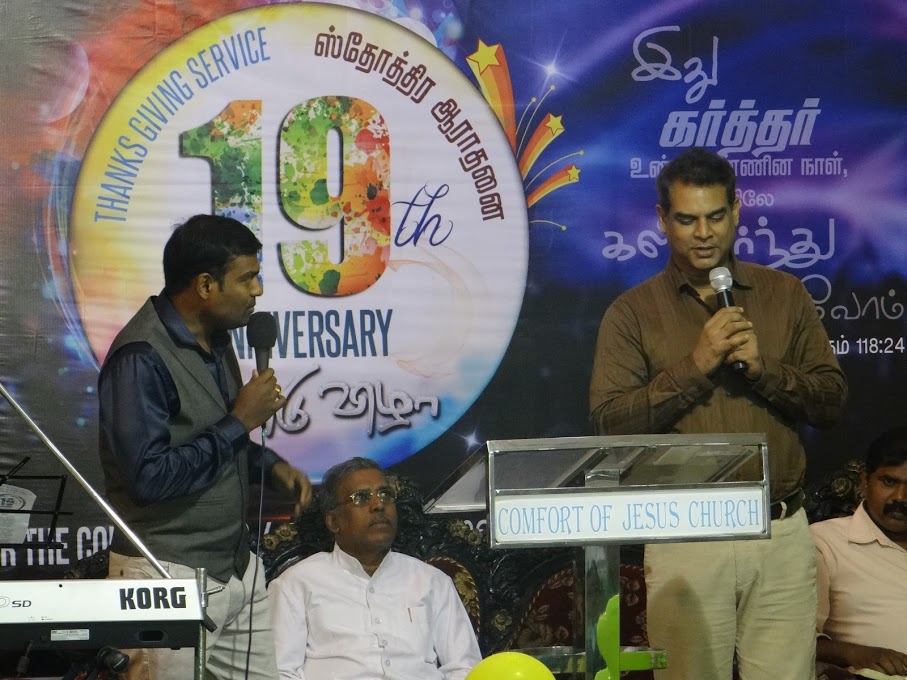The photograph captures a sermon at Comfort of Jesus Church, vividly displaying a significant event. The image features four men. From left to right: 

- A man with black hair stands holding a microphone.
- A man in a white collared shirt sits calmly.
- A podium prominently bearing the church's name in blue font on a white background separates the first two men from the next.
- To the right of the podium stands another man, dressed in a brown shirt and holding a microphone.
- Finally, another man sits, wearing a beige collared shirt.

The setting is accentuated by a tall, visually striking banner in the background. The banner prominently reads "Thanksgiving Service" and "19th Anniversary," with the number "19" displaying a dynamic paint splatter effect. The rest of the background is purple, adding to the vibrant atmosphere. The scene is detailed with elements of a religious ceremony, and subtle indications, such as Middle Eastern script, suggest a multicultural context. Both standing men are nicely dressed, with attention to detail such as the black belt and long-sleeved shirts, emphasizing the formality of the occasion.